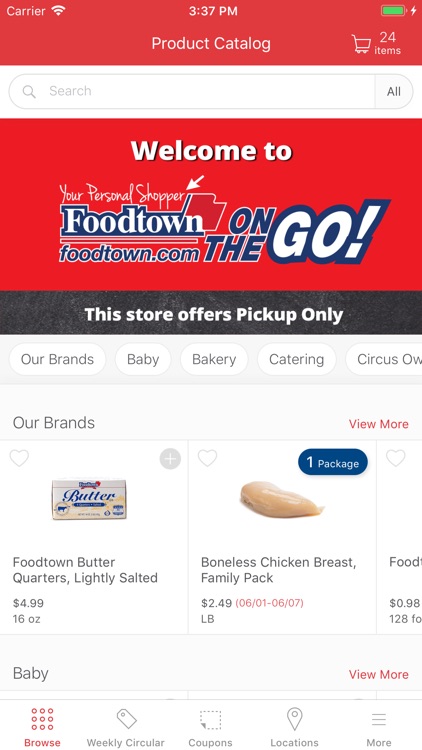In this image, it appears that someone took a screenshot of their phone while browsing a shopping app. Here is a detailed breakdown of the elements visible in the screenshot:

1. **Top Banner:**
   - The top of the screen features a light red banner.
   - On the top left corner, the word "carrier" is displayed in white, alongside the Wi-Fi connectivity symbol.
   - In the middle, the time "3.37 PM" is shown.
   - Below the time, the text "Product Catalog" appears.
   - To the right, there's an icon of a shopping cart with the text "24 items" next to it.

2. **Search Bar:**
   - Below the red banner, there's a smaller white banner running from left to right, containing a search box with a diagonal magnifying glass icon.

3. **Welcome Banner:**
   - Another red background section follows, featuring the text "Welcome to" in thicker white font.
   - Directly below the "O," a white arrow pointing to the left is visible, with the text "Your personal shopper" in cursive white font.

4. **Branding Section:**
   - Below the welcome message, the logo "Foodtown" appears. The letters are white with a blue outline.
   - Underneath the logo, two small white lines are shown, followed by the text "foodtown.com" in blue letters with a white outline.

5. **Slogan:**
   - To the right of the logo, the text "On the go!" is displayed prominently:
     - "On" is written in blue with a white outline.
     - "The" is displayed below "On."
     - "Go!" is the largest, in white letters with a blue outline.

6. **Pickup Information:**
   - A gray banner provides additional information, stating "This store offers pickup only" in small white font.

7. **Featured Products:**
   - Below the gray banner, the background turns white, displaying two product images:
     - "Foodtown Butter Quarters, Lightly Salted"
     - "Boneless Chicken Breast Family Pack"
   - These are clickable items for ordering food for pickup.

This comprehensive description highlights the various elements of the screenshot, providing a clear and detailed caption for the image.